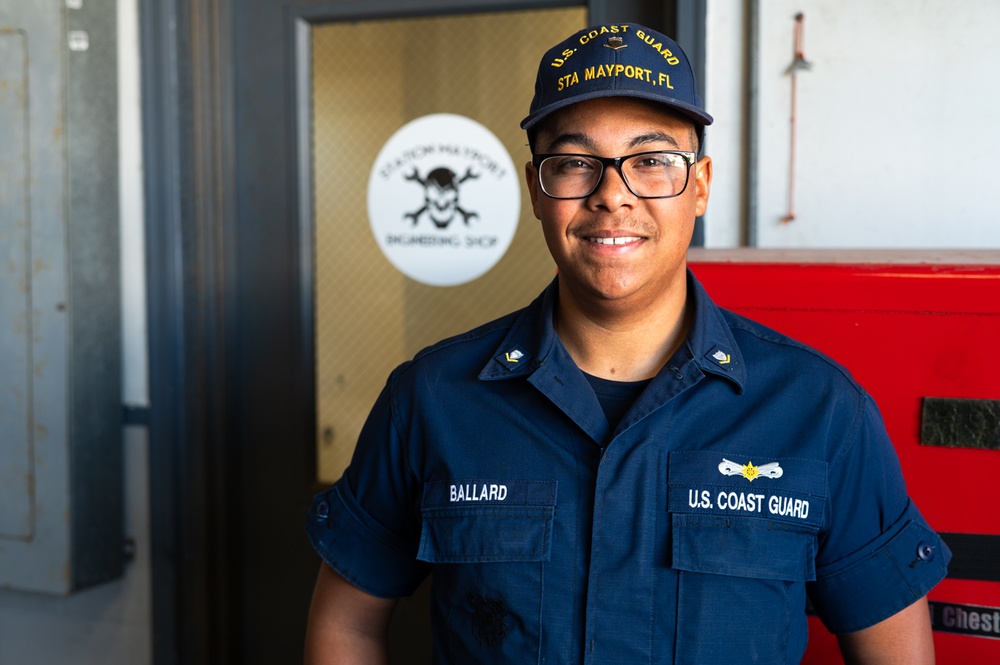This photograph features an African-American U.S. Coast Guard serviceman standing inside what appears to be a service garage or maintenance area. He is wearing a navy blue Coast Guard uniform, with the name "Ballard" embroidered over the right breast pocket and "U.S. Coast Guard" along with its logo over the left breast pocket. He is also sporting glasses and a cap that reads "U.S. Coast Guard STA Mayport, Florida" with an additional logo above the brim. Behind him is a white wall with a door that has a skull and crossbones emblem on its glass window, suggesting restricted access. To his right, there is a red toolbox-like structure and above it, a section of the white wall. Additionally, a slightly rusty, gray fuse box is visible on the far left side of the image. The photograph captures the serviceman in the midst of a work environment, exuding readiness and professionalism.